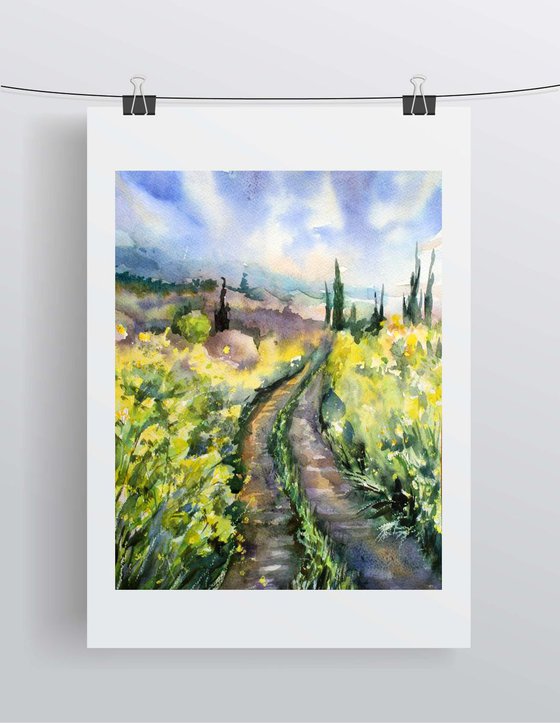This watercolor painting hangs against a white wall, suspended by a black string fastened with two paper binding clips. The painting depicts an outdoor scene featuring a winding road that extends from the bottom towards the right side, set against a grey and white backdrop. The road is depicted in a blend of brownish-beige or brownish-orange and purple hues, with green grass growing in the center, a common sight on lesser-traveled paths. On either side of the road, green and yellow flowers bloom amidst a grassy field. The background showcases a blue sky with white clouds, and off in the distance, one can see tall, thin columnar trees to the right and a mountainous landscape to the left.